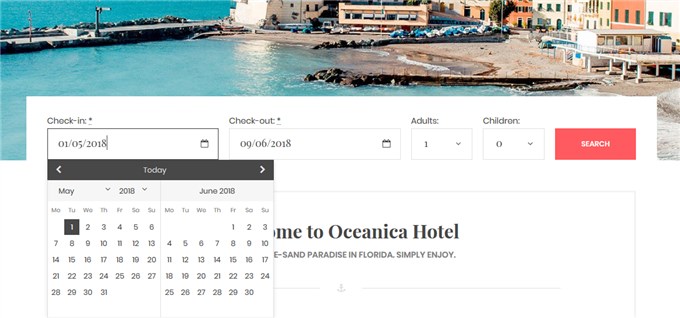This image depicts a comprehensive app interface designed for booking hotel stays, specifically spotlighting the luxurious Oceanica Hotel in Florida, a veritable paradise. At the top of the app's interface, a panoramic image captures the scenic surroundings of the hotel. The left half of the image showcases a tranquil expanse of water dotted with boats, while the right half displays an urban vista complete with towering buildings and a pristine beach, highlighting the diverse attractions near the hotel.

Below the image, there is a functional white section where users can manage their bookings. This section features interactive fields for "Check-in" and "Check-out" dates, each accompanied by a handy drop-down calendar to streamline the date selection process. Adjacent to these date fields, there are input options for specifying the number of adults and children, allowing for tailored accommodation searches based on the user’s specific requirements. Once the necessary details are entered, users can initiate a search to find available hotel rooms that match their criteria, ensuring a seamless and customized booking experience.